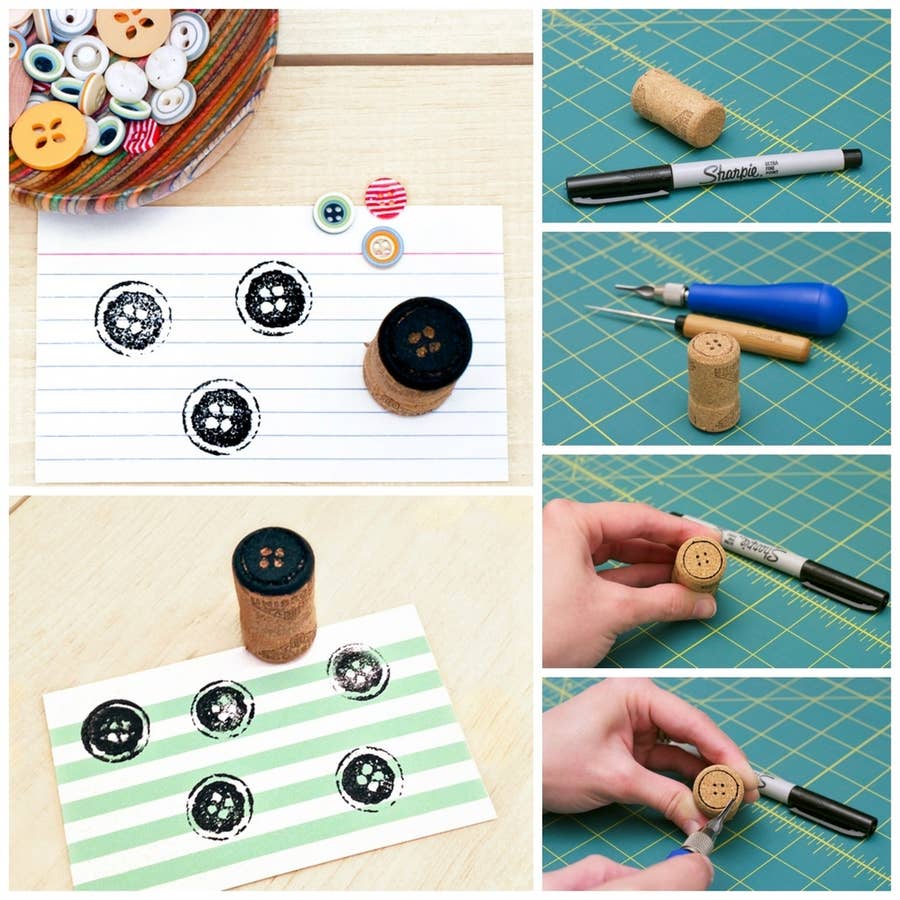The image appears to be a detailed guide on creating DIY button stamps using a spool and Sharpie marker, set within an instructional or informational website for crafting projects. The left side prominently features two images: on top, a padded fabric piece holding a variety of buttons in colors such as white, green, yellow, and red stripes next to an index card with three black spool-top stamps and three buttons lying beside it. Below this, there's another green-and-white-striped index card displaying five black spool-top stamps. On the right side is a step-by-step sequence showing the creation process: the first image shows a spool and a Sharpie pen, the second depicts the spool with a couple of wooden-handled tools, the third focuses on a hand holding the spool with the Sharpie nearby, and the last image shows someone preparing to draw on the spool with the Sharpie. This visual guide is set against a wooden table, with a bowl of multi-colored buttons placed near the top image, all designed to illustrate the process of transforming a spool into a functional button stamp.